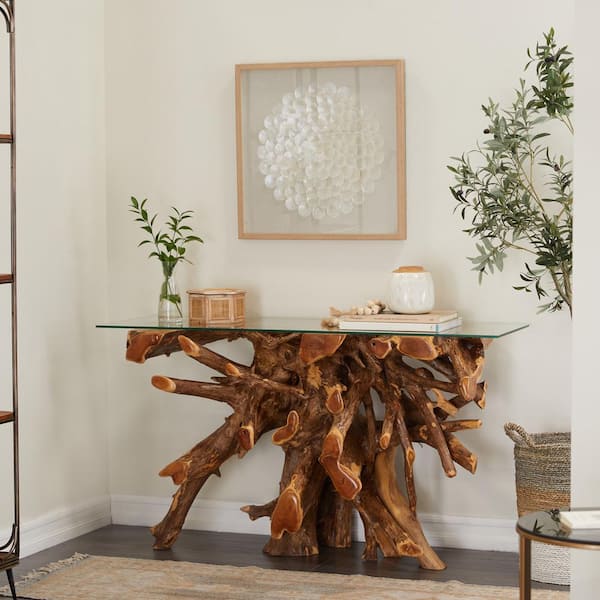The image is an indoor scene, likely a living room, showcasing a stylish and well-decorated space with a white wall and white baseboards. The floor is a sleek gray, complemented by a tan rug. To the left, there's a partially visible multi-section wooden shelving unit in brown. In the lower left, a wicker basket can be seen. Centered on the back wall is a large piece of artwork with a beige-gray hue and a circular pattern, framed in light wood. 

The main focal point is a unique rectangular glass table up against the wall. The table’s support structure is crafted from bunches of tree branches arranged in a wild, natural pattern. On the table are several decorative items: a glass container with green leaves, a white vase, a round shiny container, a porcelain jar, and a couple of books. In the lower right of the image, there's a round end table with brown legs, and nearby, part of a plant with branches and green leaves is glimpsed, adding a touch of nature to the decor. The overall color palette of the room includes accents of brown, green, white, and tan, creating a harmonious and inviting atmosphere.